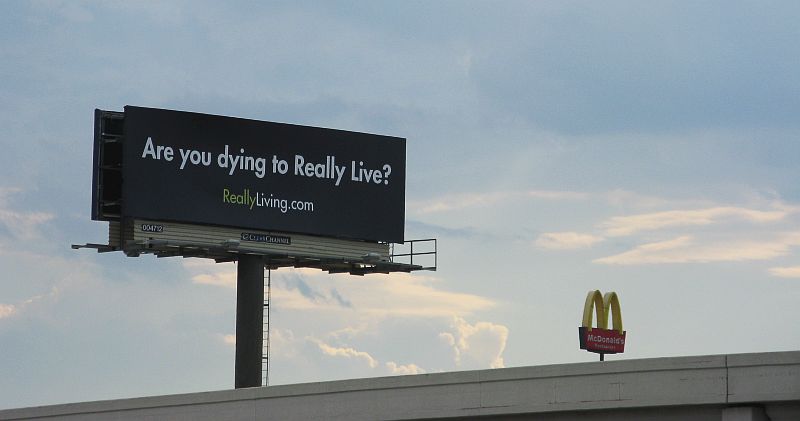This photo captures a scenic view from a car on a freeway overpass. Dominating the scene, a large rectangular billboard rises against an expansive, sky-dominated background. The sky is a mix of bright blue with occasional white clouds, suggesting a clear day. The focal point, the billboard, features a striking black backdrop with bold white text asking, "Are you dying to Really Live?" The words "Really" and "Live" both start with capital letters. Below this message, in smaller text, is the URL "reallyliving.com," where "really" is highlighted in green. Adjacent to the billboard, the iconic golden arches of a McDonald's sign are visible, with the familiar red banner displaying "McDonald's" in white text. The billboard stands on a sturdy concrete pole equipped with a ladder, hinting at its significant height. The scene conveys a blend of commercial and urban elements set against a tranquil sky.